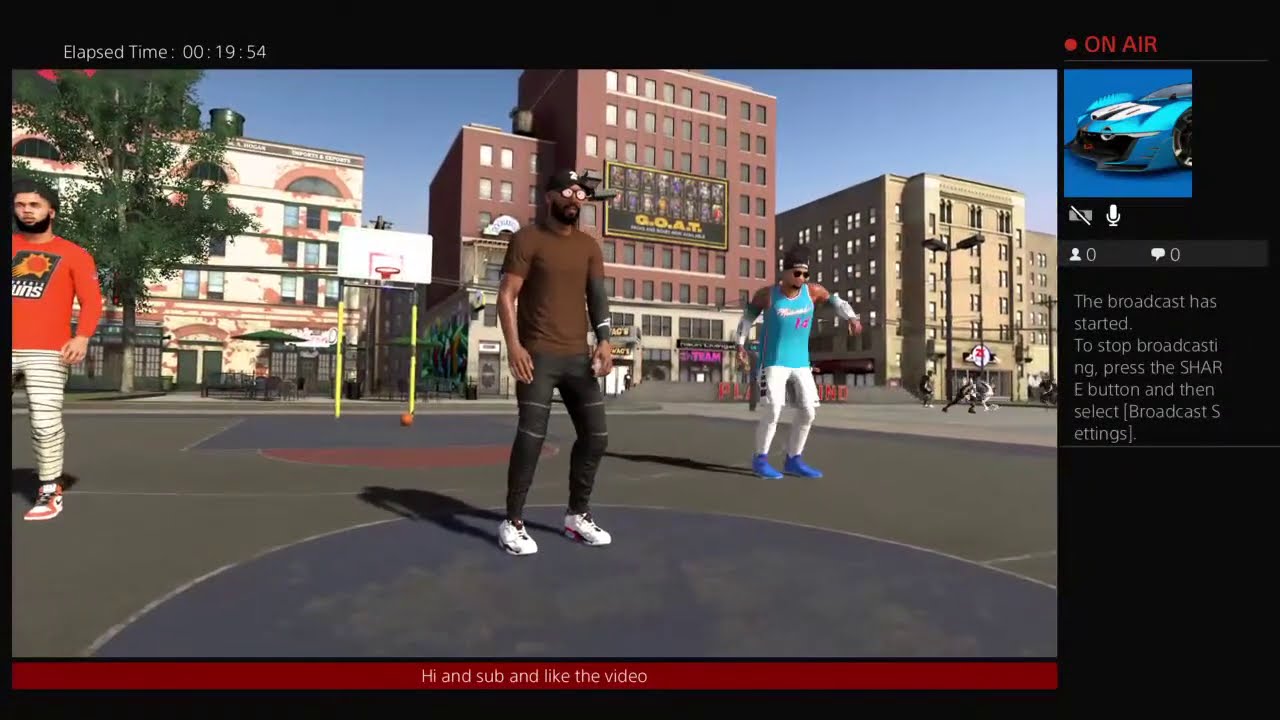The image is a still from a video game, likely part of the 2K series, showing three characters standing on an outdoor basketball court in a city setting, with buildings ranging from four to eight stories in the background. The characters are rendered with a blocky, computer-generated appearance. 

On the left is a character with a beard, black hair, and a red Phoenix Suns shirt, paired with white pants featuring black stripes, and red Nike shoes. In the middle stands another character wearing a brown shirt, black pants, white sneakers, an arm sleeve, a black hat, and glasses. This central figure seems to be the focal point of the image. To the right is a character dressed in a teal jersey, white pants, and blue sneakers.

The court scene shows aspects of an urban environment and suggests the game is about to start, as indicated by the players' readiness and slightly animated stances. The image includes a visible basketball and hoop, and other players can be seen in the background. Additional on-screen elements indicate it's a streamed game with streaming interface details such as "on-air" status, elapsed time counter, and prompts for audience interaction at the bottom of the screen.